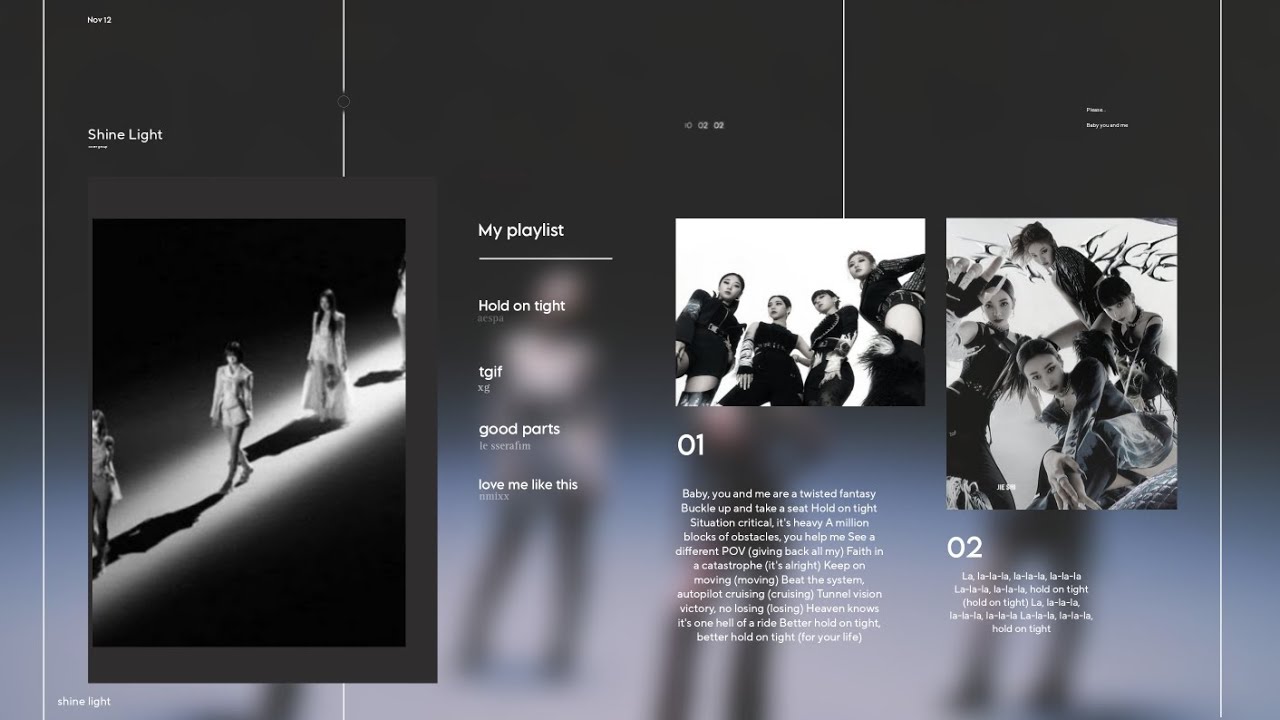In this vividly designed music platform interface, the background transitions from a light gray and blue gradient at the bottom to a rich dark gray and black at the top. On the left side of the image, there's a dark gray framed photo depicting four people walking down an illuminated aisle. Adjacent to this image, a series of categories are listed: "My Playlist," "Hold On Tight," "TGIF," "Good Parts," and "Love Me Like." To the right, there are two additional images. The first is a white-bordered photograph of four band members standing side by side. Below this image, the label "01" appears, followed by a paragraph of tiny white text. The second image to the far right is a black and white photo featuring four band members posing for the camera, with the label "02" and another block of small white text below it. In the top left and top right corners of the image, small white text is present, adding to the intricate detailing. Enhancing the structure and symmetry of the layout, four thin vertical white lines are positioned: one on the left, one on the right, and two at the top, completing the meticulously designed interface.